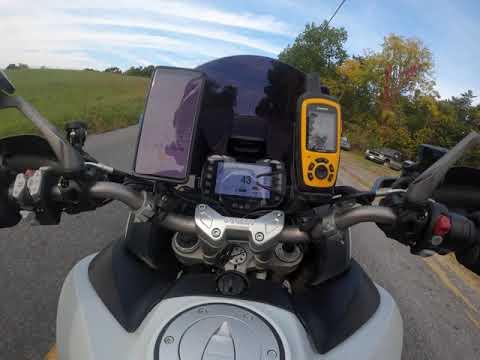The image captures an outdoor scene from the perspective of someone seated on a motorcycle, likely paused on a country road. The focus is on the motorcycle's gray body, black handlebars, and gray brakes. Mounted on the dash are various devices, including a cell phone on the left, possibly a GPS or satellite phone in the center, and what seems like a walkie-talkie on the right. The road, paved and gray, shows a hint of a yellow line. Surrounding the road are green expanses—a grassy area to the left and a row of trees with both dark and light green leaves to the right, under which a pickup truck and another car are parked. Above the trees, power lines stretch across the top, set against a bright blue sky adorned with feathery white clouds.